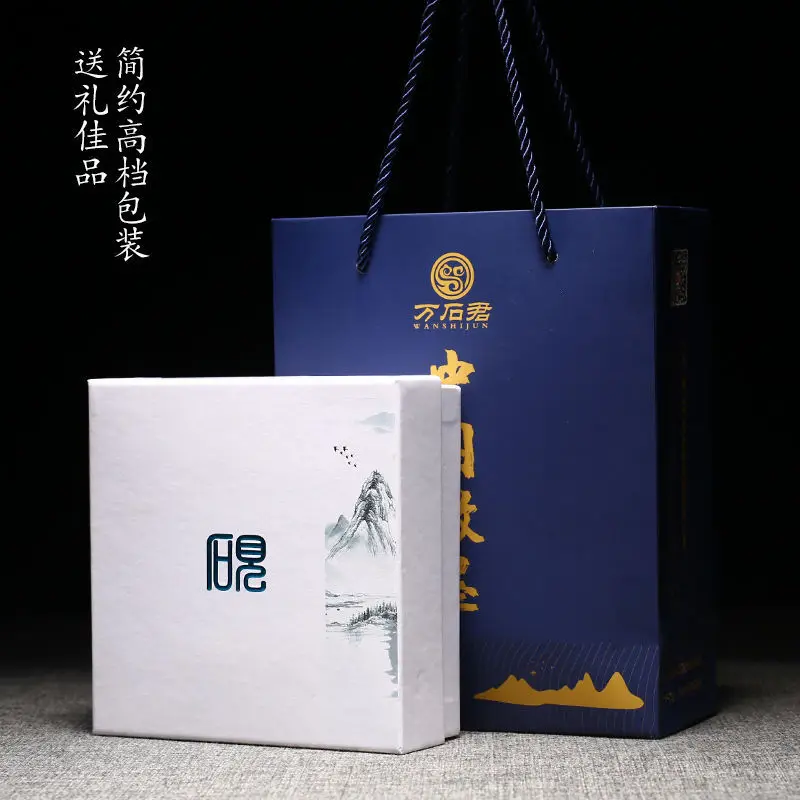In the foreground of the image, against a mainly black background, a white package sits on a gray carpeted or felt floor. The package features a dark blue logo in the center that resembles an Allen wrench, an upside-down "A" next to an "S", and a grid. On its right side, there are black-and-white stencils of mountains with trees beneath and a river or lake. Behind the package stands a dark blue, vertical rectangular gift bag with dark blue strings serving as handles. This bag is adorned with gold Japanese or Korean text running down its middle and a gold mountain range in the bottom right corner. In the upper left corner of the image, against the black background, there are two vertical columns of white Japanese text.